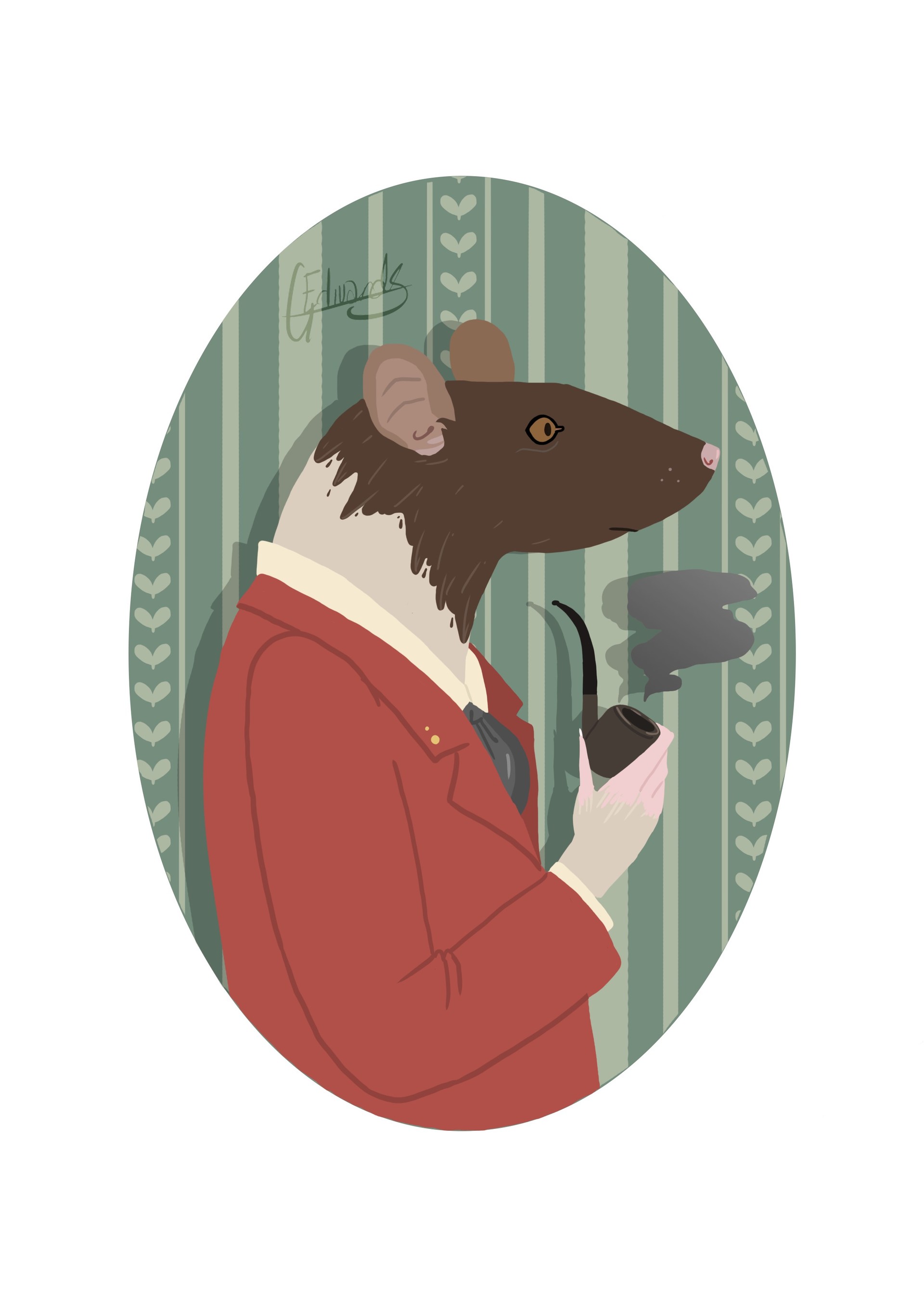This image features an oval-shaped painting set against a white background, framed by a green and white striped wallpaper. The wallpaper's stripes alternate between light and darker green, with the darker stripes adorned with small off-white hearts, arranged vertically along the leftmost, rightmost, and center stripes.

The painting, executed in a cameo-style reminiscent of early 1900s portraits, depicts a brown mouse with a pink nose and tan-colored ears. The mouse, dressed in human attire, is wearing a muted red suit jacket over a white dress shirt with a black tie. It stands upright, holding a smoking pipe, which is black with a charcoal gray front. A small tuft of gray smoke rises from the pipe.

Adding to the detail, the mouse has a long snout, brown eyes, and human-like hands. It is positioned in profile, facing to the right, giving the image an absurdist, almost cartoon-like quality.